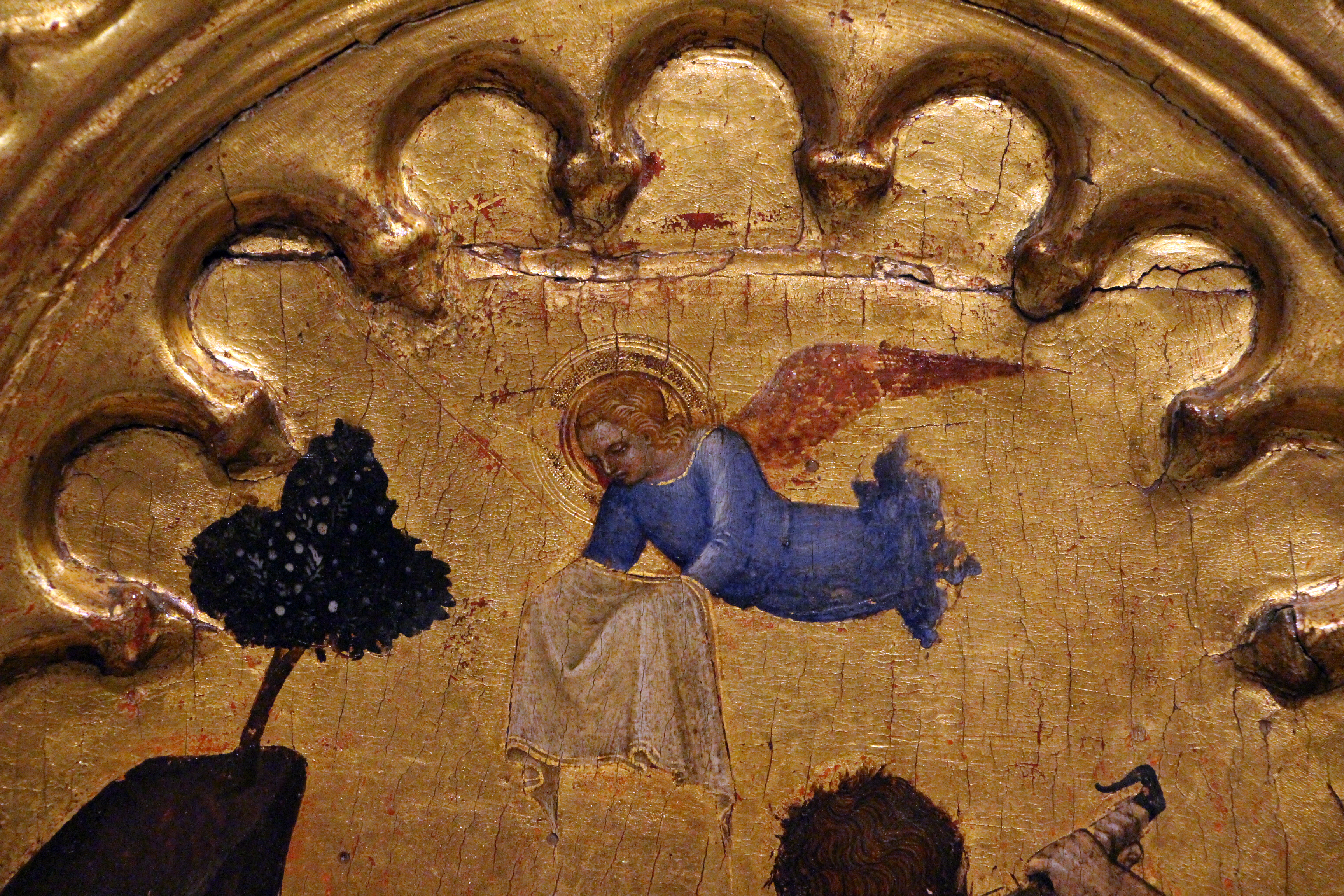This image, likely a photo of an icon or oil painting set in a religious context such as a cathedral, features a serene angel adorned in a vibrant blue robe, floating gracefully within a golden, scalloped archway. The gold leaf backdrop, though aged and cracking, accentuates the ethereal and timeless quality of the composition. The angel looks downward with a calm, contemplative expression, her reddish-brown wings contrasting against the iridescent gold. She holds an off-white towel draped over both hands. To her left, a tree rises from a hill, adding a touch of nature to the celestial scene. Below the angel, there appears to be a partially visible round figure, perhaps a head, adding a sense of mystery and depth to the image. The intricate border resembles interlocking arch-like extensions, framing this celestial and serene moment beautifully.